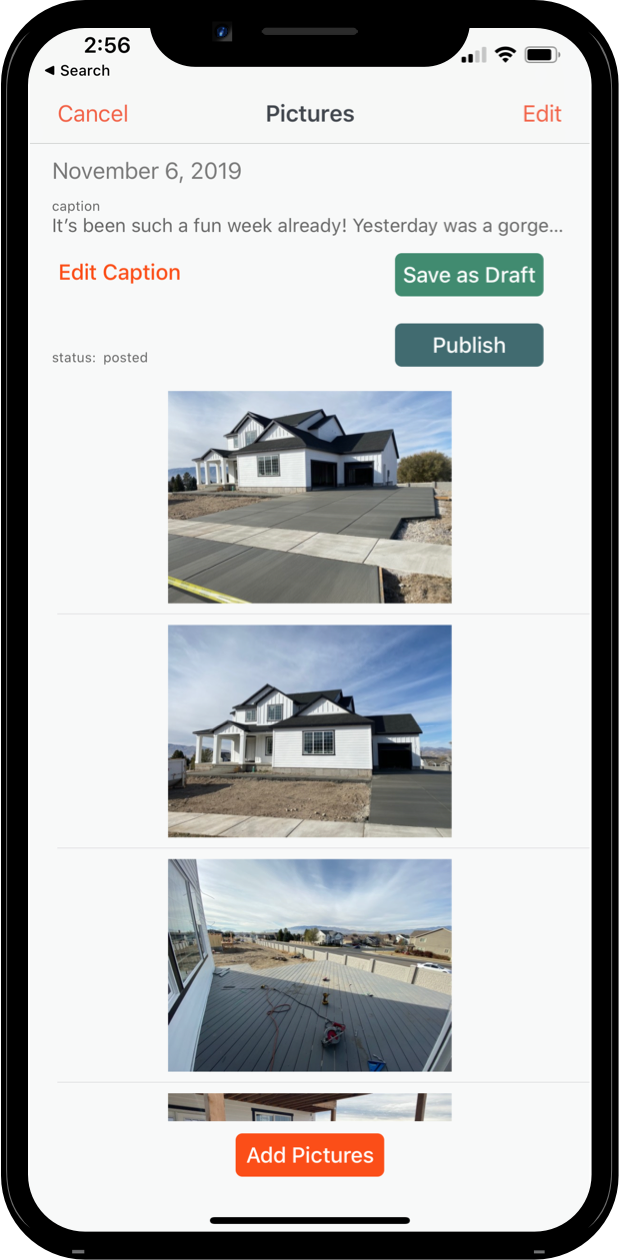A comprehensive image of a smartphone screen reveals various interface elements. At the top-left corner, the time reads 2:56, with "search" displayed below it. On the top-right corner, service and Wi-Fi indicators are present alongside a battery icon. Directly beneath this status bar, the interface displays options for navigating with "cancel" on the left, "edit" on the right, both in orange text, and the word "pictures" situated in the center.

Further down, in gray text, the date "November 6, 2019" is shown, followed by an incomplete caption that reads, "It's been such a fun week already, yesterday was gorge..."—with the word "gorgeous" likely being cut off. Below this caption, instructions for "edit caption" are highlighted in orange text. A green button labeled "save as draft" in white text appears to the right, and a darker greenish-blue button beneath it reads "publish," also in white text. The phrase "status posted" is displayed in gray to the left of these buttons.

The bottom of the screen showcases images of a newly constructed house, featuring a white exterior with contrasting gray and black roofs. A closer inspection of the images, particularly the third one, reveals construction tools and yellow tape, suggesting the house is still under construction. Additionally, there is no lawn present, only dirt and a visible concrete foundation, reinforcing the notion that the construction is still ongoing. The layout shows three distinct pictures of the house, while a fourth image is partially visible, cut off at the edge of the screen.